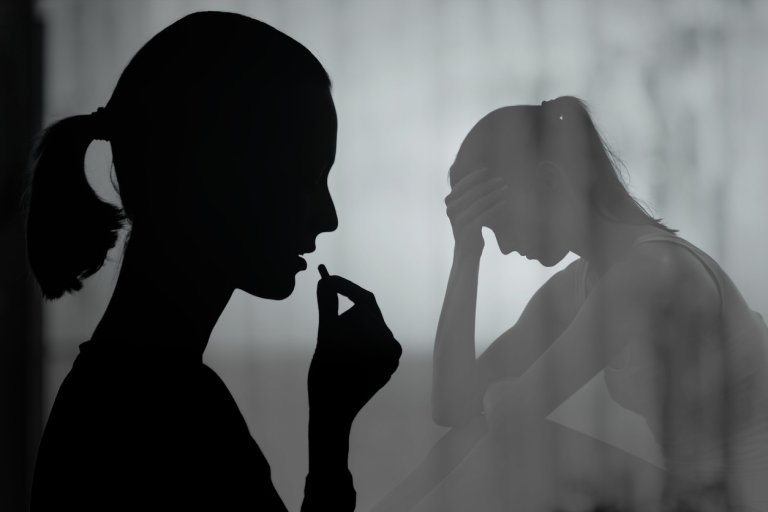The image portrays a dual representation of the same girl, split into two sides. On the left side, there's a dark, 2D outline of the girl rendered in deep black, depicting her with a short ponytail and a thin neck. She is holding a pill in her left hand, appearing to prepare to take it. On the right side, a more three-dimensional, grayscale depiction of the girl sits with her head bowed, her right hand pressed to her forehead in a gesture that conveys deep distress or depression. She is dressed in a tank top and has her hair in a longer ponytail. The background is a blend of gray shades, accentuating the somber, reflective mood of the image. Both representations, left and right, face each other, suggesting an internal conflict or duality within the same person.